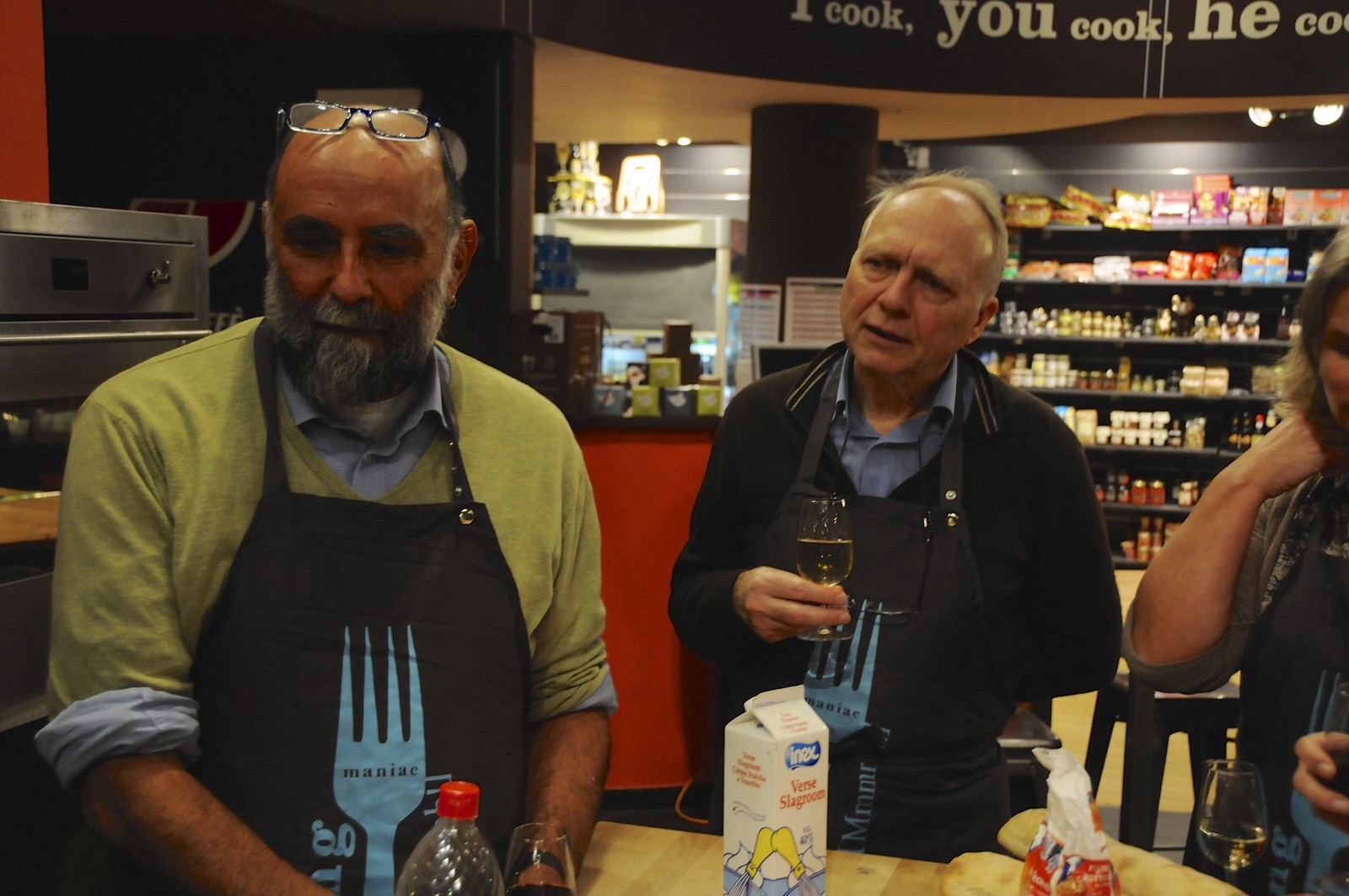The image captures a scene inside what appears to be a restaurant, grocery store, or coffee shop featuring two men and a woman on the right. The setting has black shelves filled with assorted food items in the background, and a counter area on the left side that looks like a place to pay. 

In the foreground, there's a wooden table. The man on the left is seated and wears a lime green shirt with a black apron featuring a blue fork and the text "maniac" printed on it. He has a thick black and gray beard, glasses resting on top of his balding head, and his shirt sleeves rolled up to his elbows. In front of him, there's a red capped bottle and a wine glass. 

To his right is another older man, also bald but with more visible gray hair. He wears a black jacket over a blue shirt and a similar black apron. He holds a half-filled wine glass containing a light yellow drink, and in front of him, there is a milk carton labeled "Verslagroom." 

The woman on the far right is partially visible, with shoulder-length dark brunette hair. She appears to be adjusting the shoulder strap of her apron and has a wine glass in front of her as well. 

The detailed background and presence of various drinks suggest a food or wine-tasting event.